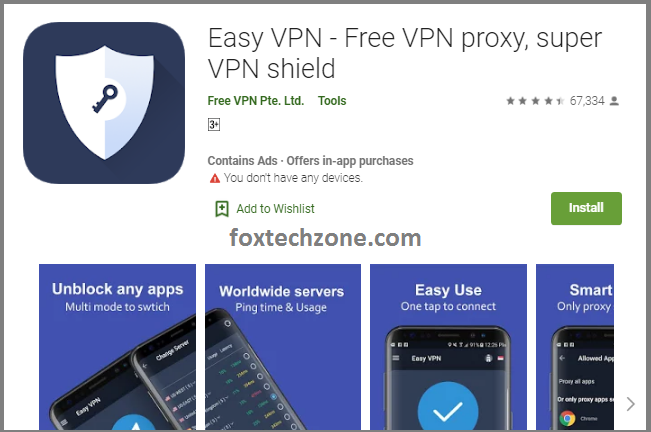The image is a screenshot of an Apple Store page displaying the "Easy VPN - Free VPN Proxy, Super VPN" app. At the top left corner, there is the app's icon, followed by the title "Easy VPN - Free VPN Proxy, Super VPN." Below the title, in small green text, it says "FREE VPN PTE. LTD." and "Tools." On the right side, there is a rating of 4.5 out of 5 stars, along with the number of reviews, "667,334," and a user icon.

Under the "FREE VPN PTE. LTD." label, there's a box labeled "3+," indicating the app's age rating. Below that, in light gray text, it says "Contains ads · Offers in-app purchases." Further down, there's a red triangle with the message "You don't have any devices" in gray text. Next to it, a green plus flag symbol is accompanied by the text "Add to Wishlist" in green. Below this, "foxtechzone.com" is displayed in gray.

On the right side of the screen, there's a green "Install" button with white text. Beneath this are four screenshots of the app in use. The first screenshot highlights "Unblock Any Apps Multi Mode Switch," the second showcases "Worldwide Service Ping Time and Usage," the third advertises "Easy Use One Tap to Connect," and the fourth, partially visible, mentions "Smart Only Proxy." All four screenshots feature images of phones displaying the app's interface.